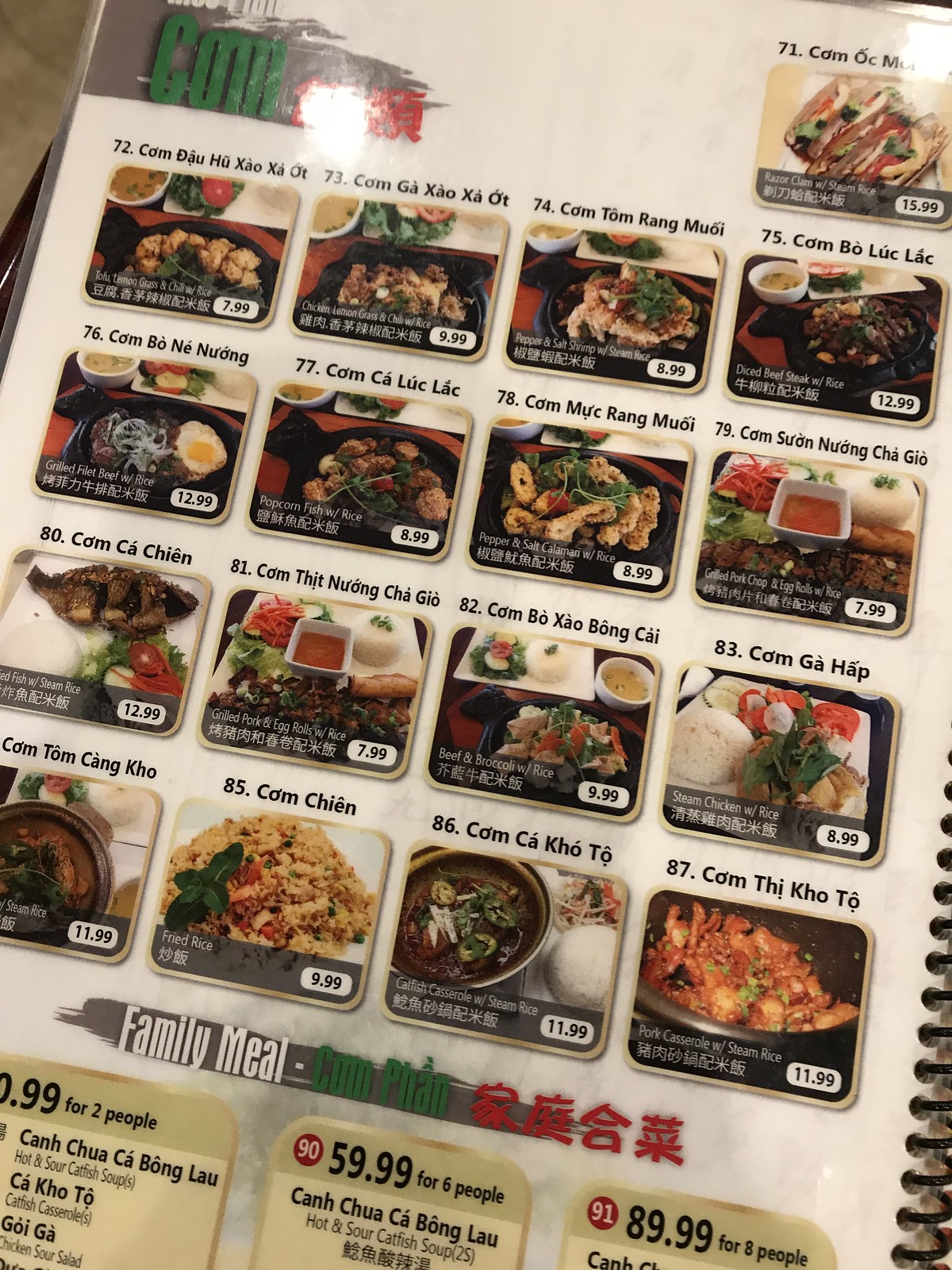The image depicts a laminated menu printed on white paper with a plastic covering, giving it a glossy sheen. The menu is bound by a black spiral running from the bottom right corner halfway up the right side. The menu is slightly tilted to the right, and in the upper left corner of the image, part of the taupe-colored floor is visible.

In the upper left corner of the menu, the text "COM" is printed in green on a gray background, alongside red Chinese characters. The menu features several rows of dishes, each marked with specific numbers. 

In the first row, starting from the upper right corner, the menu lists:
- Number 71: Razor clams with rice.

The subsequent rows list the following dishes:
- Second row: Numbers 72, 73, 74, and 75.
- Third row: Numbers 76 through 79.
- Fourth row: Numbers 80 through 83.
- Fifth row: Numbers 84, 85, 86, and 87.

Below these rows, on a gray stripe, the phrase "FAMILY MEAL" is written in white letters, followed by "COM PAN" and more Chinese characters. 

The family meal options are listed with pricing for various group sizes:
- $29.99 for two people, including hot and sour catfish soups, catfish casserole, and chicken sour salad.
- $59.99 for six people (listed as dish number 90) includes hot and sour catfish soup.
- $89.91 for eight people (listed as dish number 91).

The detailed description of menu items, pricing, and the layout provides a clear and comprehensive overview of the image.